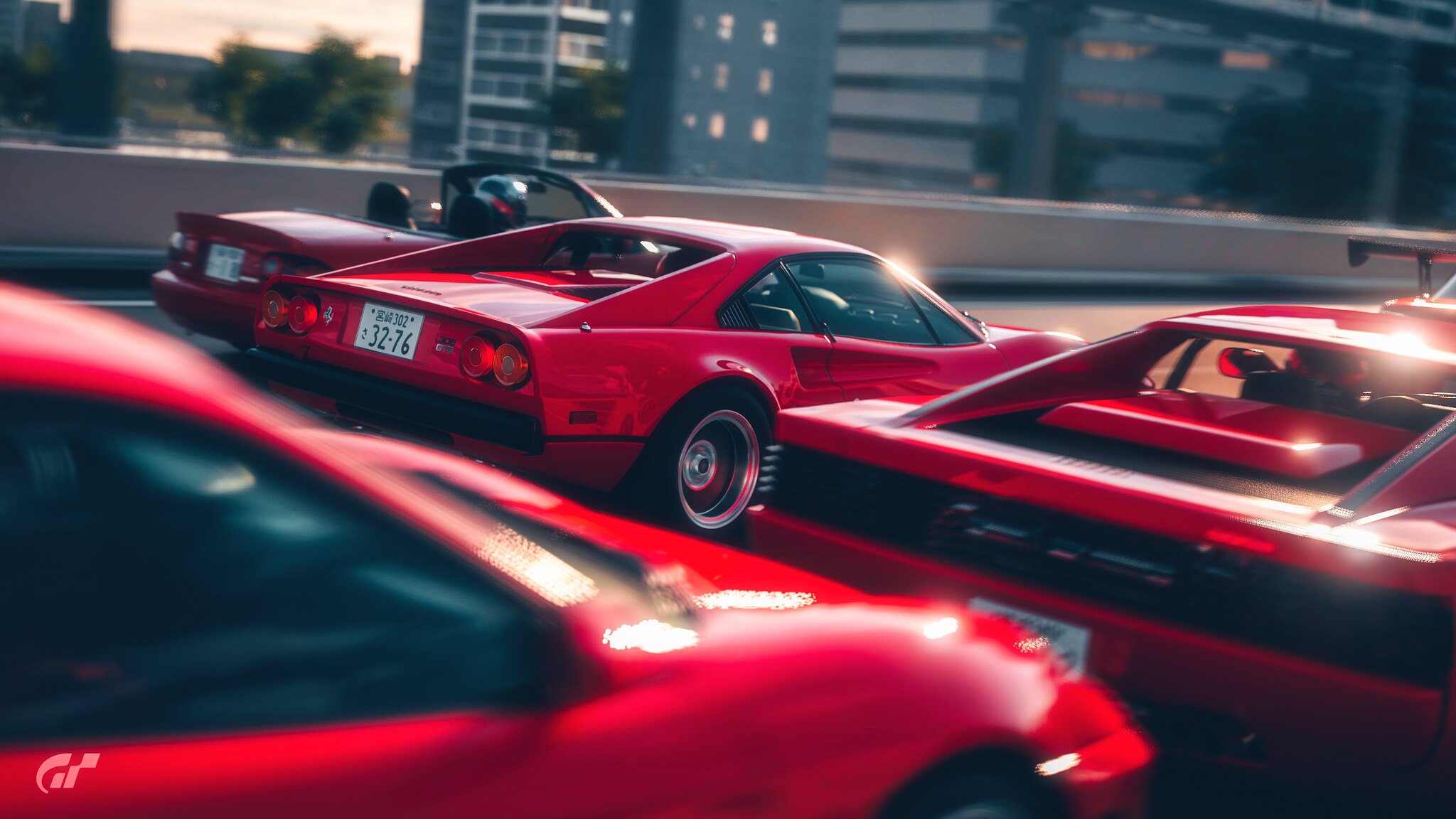This dynamic landscape-oriented photograph captures a vivid, red-themed scene on a bustling street, likely depicting expensive sports cars either in motion or poised to race. The image centers on four striking red vehicles, each exuding high performance and luxury. To the far left, a sleek convertible, possibly a Triumph, showcases its sporty appeal with the top down, revealing a driver wearing a racing helmet. Adjacent to it is a sophisticated Maserati-like sports car, noted for its impressive black tires and the reflective shine on its bodywork. The third car in the sequence, resembling a classic Charger but with square headlights, also dons a racing helmet-clad driver visible through the back window, with sunlight gleaming off its roof. The final vehicle, partially obscured, appears in the background with only its red roof, hood, and a section of a darkened window visible, adding a sense of motion and depth to the scene.

The backdrop comprises a striking urban landscape with a mix of architectural structures. On the right side, a prominent multi-floor blue building—likely an office or parking garage—stands tall beside a residential complex featuring balconies. The top left of the frame reveals a serene sky, dotted with distant, fuzzy buildings that hint at a sprawling metropolis beyond. Anchoring the scene is a concrete barrier running along the road, which adds a partition between the vibrant street action and the towering gray skyscrapers that fill the horizon. This photograph masterfully blends elements of realism and representationalism, capturing a moment teeming with energy and high-end automotive elegance.